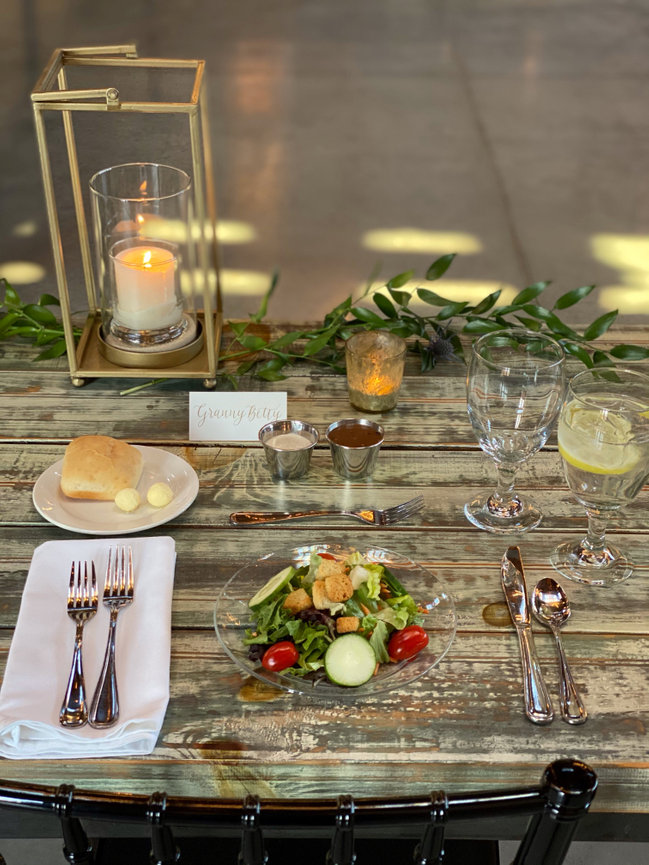The photo depicts an elegantly arranged table setting for a wedding guest named "Granny Betty." At the center of the table, a clear plate holds a vibrant salad with iceberg lettuce, cherry tomatoes, sliced cucumbers, and croutons. To the left of the plate, two forks—one for salad and one for dinner—rest on a white napkin. On the right side, a knife and spoon are positioned, with the knife on the inside and the spoon on the outside. Behind the salad plate, a small plate features a roll of bread accompanied by two butter balls. Above the plate are two small bowls filled with different dressings, one white and one red. Two glasses are placed to the right of the salad: one contains water with a slice of lemon, while the other appears empty. Additionally, the table is adorned with candles—one small and one large pillar candle enclosed in a gold frame—and a sprig of greenery adds a touch of natural decor.